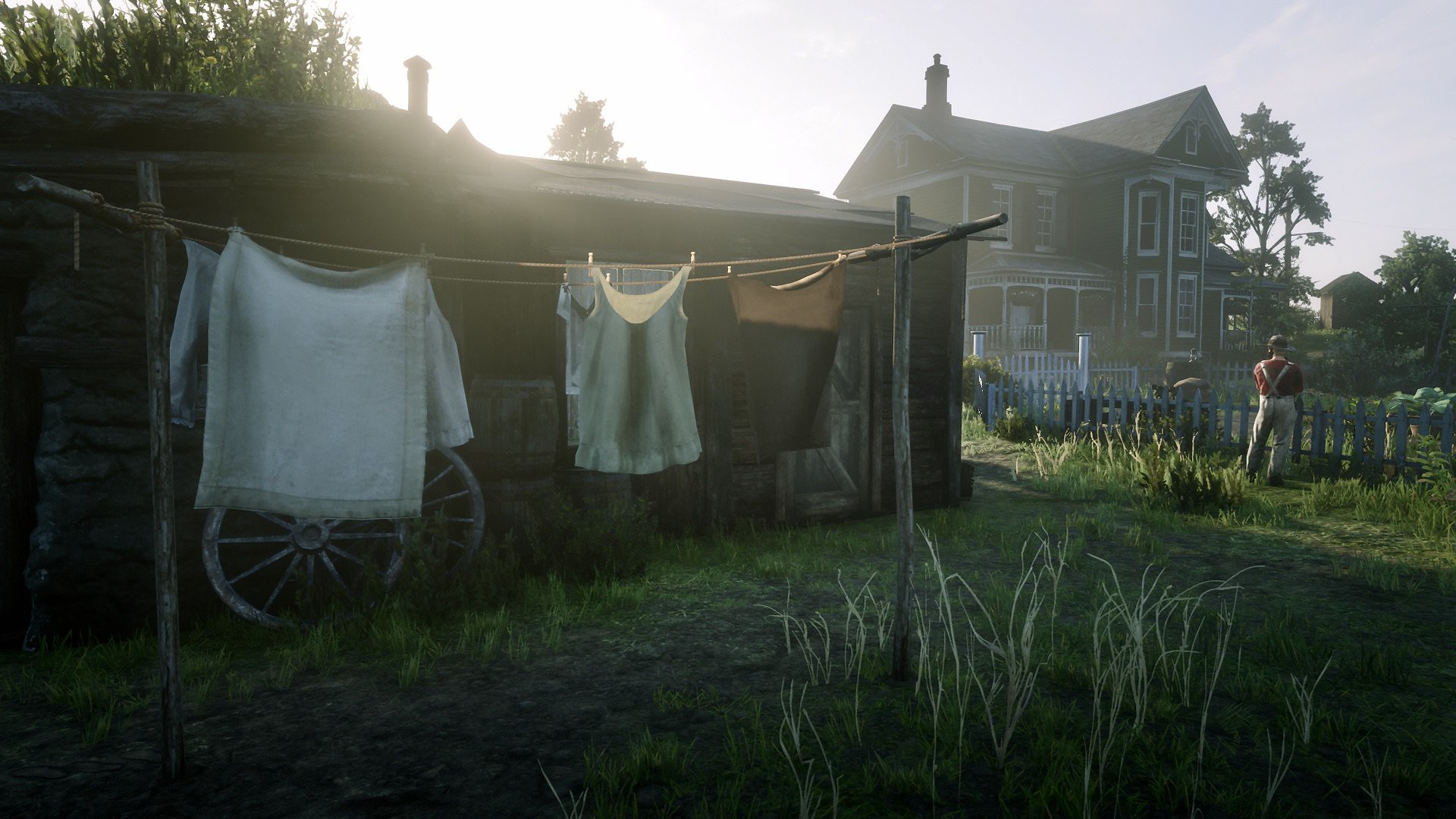In this screen capture from a video game, the scene portrays a rustic and desaturated Old West setting. Central to the image is a small shack, in front of which stands a wooden wagon with visible wheels. The top part of the scene is fairly washed out, due to the intense sunlight shining from behind the shack. To the left, an old-fashioned clothesline stretches with various rustic garments hanging to dry, reinforcing the historical feel.

In the background, a more ornate and larger house contrasts with the shack, suggesting a social hierarchy, possibly indicating that the smaller building serves as quarters for servants or workers. A man is depicted standing by a wooden fence, which seems to enclose a garden area flourishing with grass and various trees. Despite the abundant greenery, the overall color palette remains muted and desaturated, contributing to the vintage and weathered atmosphere of the setting.